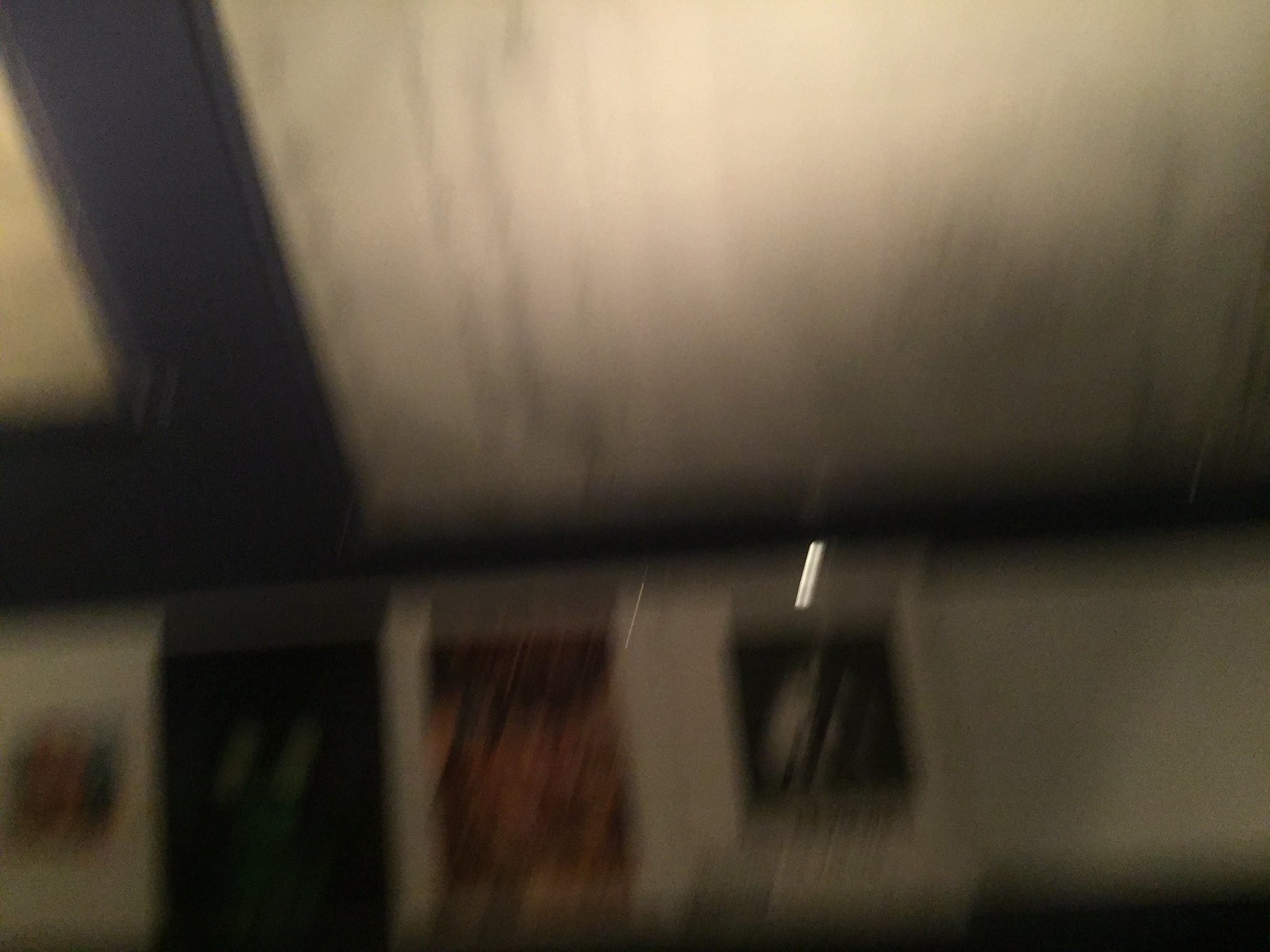This photograph is highly blurred, rendering the details nearly indistinguishable. It shows a partial view of a wall and ceiling. The wall appears to be white, though its clarity is compromised by the blurriness. The wall hosts several square, poster-like objects. The first object exhibits a mix of black, white, and a touch of green. Next, a poster-like object showcases shades of dark brown, lighter brown, and off-white. Another object is set against a black background with discernible green streaks. Adjacent to it, there is an object featuring various hues of brown, tan, and black. However, a significant light flare and general blurriness obstruct any further details from being clearly identified.